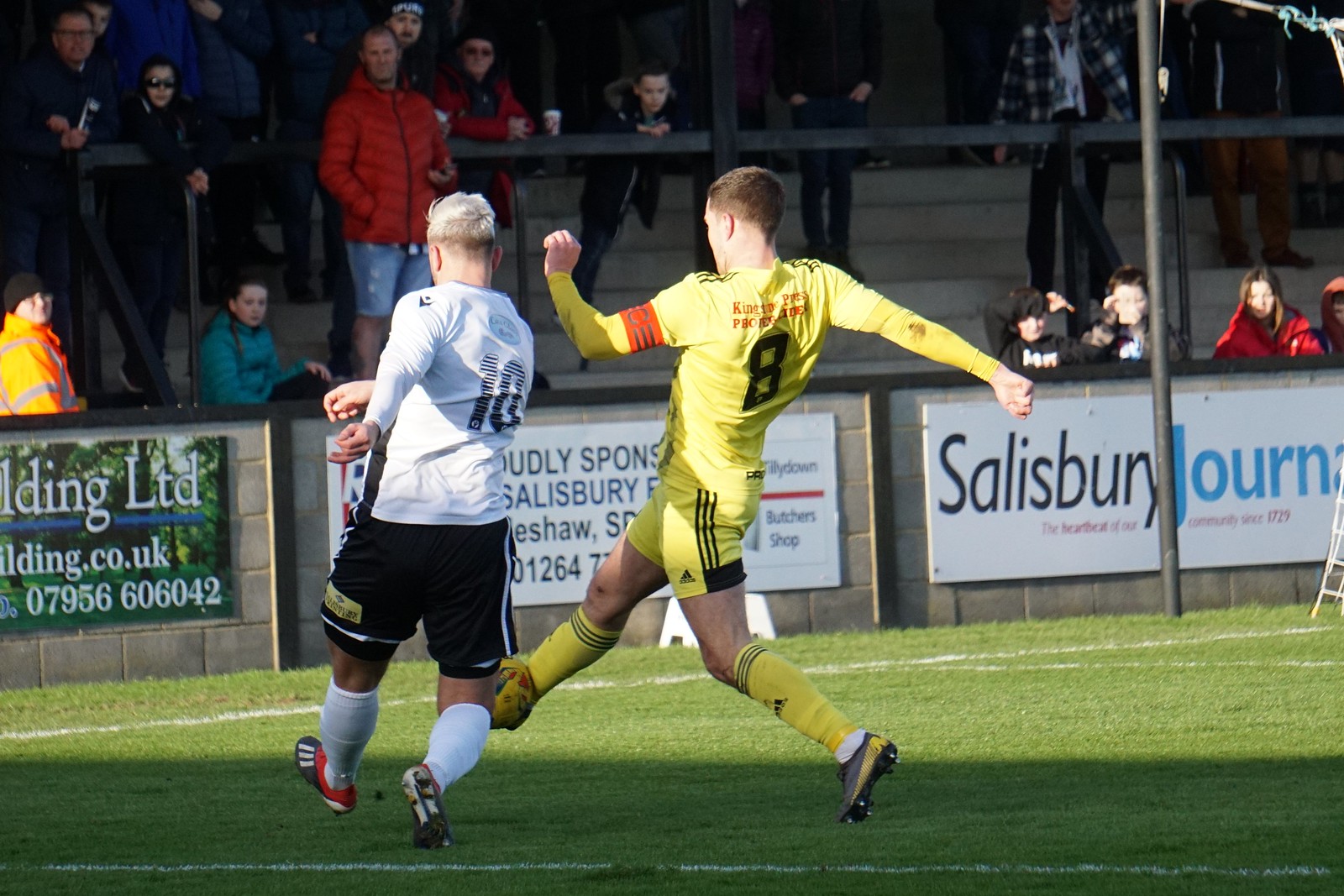The photograph captures an outdoor daytime scene of a soccer match in progress. At the center of the image, two players are captured in action; the player on the left is dressed in a white jersey paired with black shorts, while the player on the right sports a full yellow uniform consisting of a yellow jersey and matching shorts. The soccer ball is almost touching the right leg of the player in yellow, indicating an impending move.

The background features a stone wall, which functions as a boundary separating the vibrant green soccer field from the audience seating area. The seating area consists of various steps where the spectators are either standing or sitting. Multiple banners hang along the stone wall, advertising various businesses. 

To the right, a white banner with black text prominently reads “Salisbury,” followed by “Blue Text Journal,” and some illegible red text underneath. Another white banner, mostly obscured by the players, can be seen in the center. To its left, a banner showcases a printed forest background with some chopped-off white text. 

Above the banners, the audience watches intently from the stands, with a railing running along the edge to separate them from the field. There are discernable shadows cast across the lower horizontal section of the photo, indicating some overhead structures or natural sunlight creating contrast. The image is rich in colors such as yellow, white, black, blue, and various shades of green and gray, effectively capturing the vibrancy and dynamics of the soccer match.